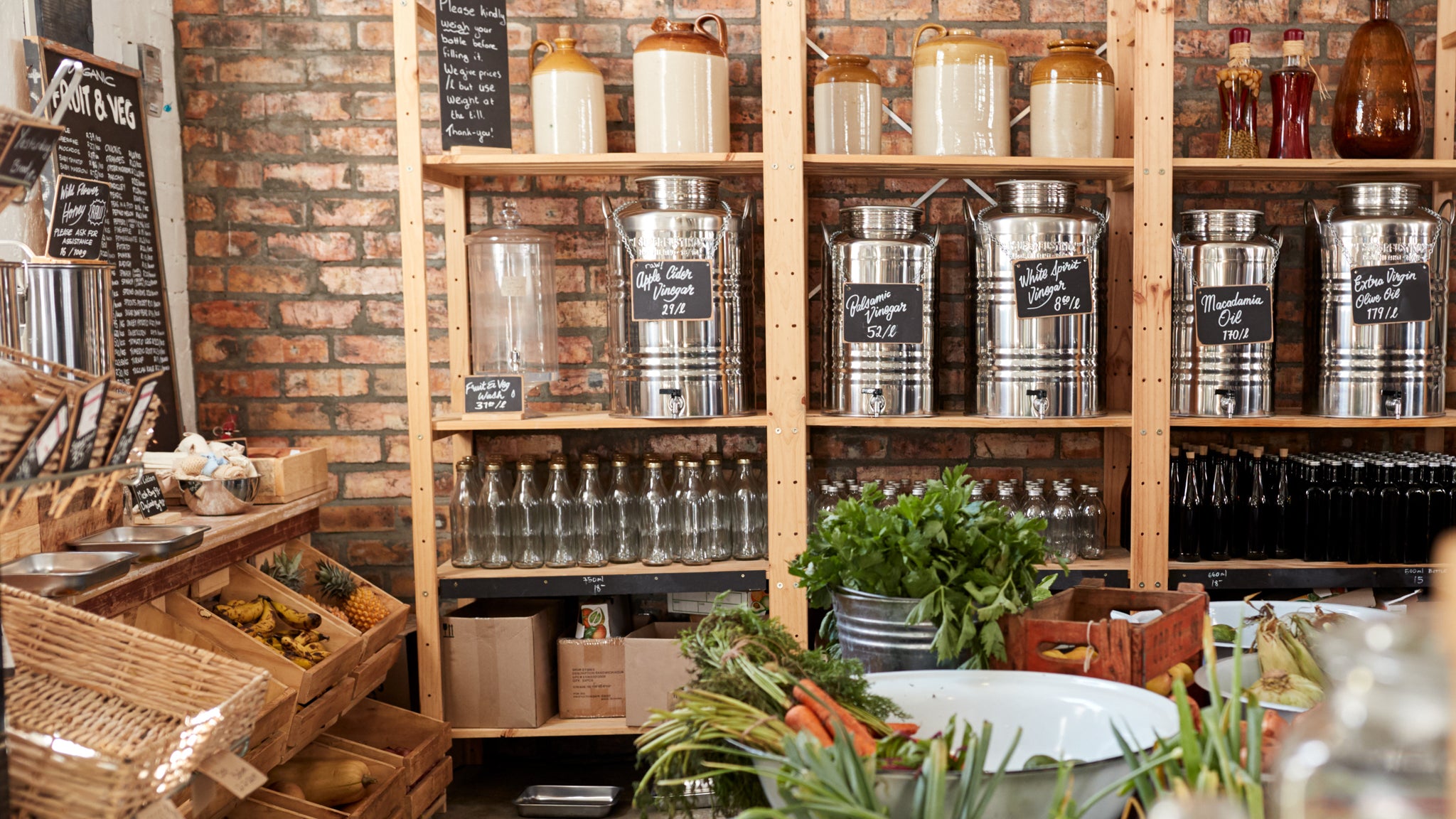This photograph appears to have been taken inside a cozy, rustic small store, possibly a coffee shop or a diner. There is a prominent brick wall in the background adorned with a shelving unit. The top shelf is lined with ceramic jugs and jars, while the bottom shelf holds metal tins and glass bottles, both clear and dark. The middle shelf features an array of labeled bottles, including apple cider vinegar, balsamic vinegar, white spirit vinegar, macadamia oil, and extra virgin olive oil. Beneath these, smaller bottles are neatly arranged, likely available for purchase.

On the left side of the picture, additional shelves and wooden crates are stacked with fresh produce, such as pineapples, bananas, and possibly squash. At the bottom, a handwritten chalkboard displays "Fruit and Veg" along with a menu or prices that are difficult to read. In the center of the setup, a table is laden with various vegetables and herbs, neatly placed in bowls and dishes. The overall ambiance conveys a charming, natural aesthetic with an emphasis on fresh, wholesome ingredients.